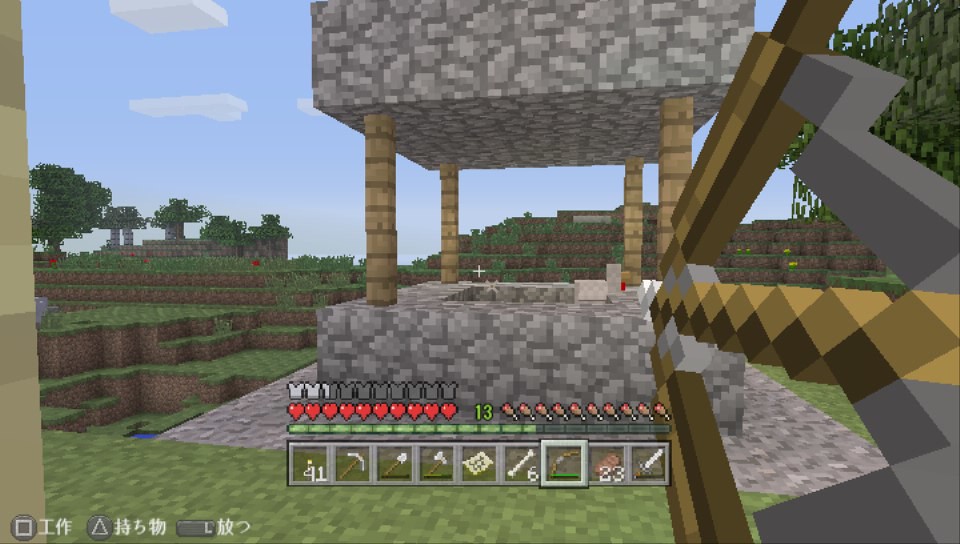A screenshot from the popular video game, Minecraft, showcasing a pixelated world under a clear blue sky scattered with a few clouds. The focal point is a square-shaped stone structure, supported by pillars at each corner. This structure stands prominently in a grassy area, with gentle hills forming the background landscape. On the left side of the image, a small patch of water is visible. At the bottom left corner of the screen, Japanese characters and various symbols can be seen. In the center, inventory slots display different tools, and a health bar with heart icons indicates the player's remaining health. Below the health bar, there's an experience meter, filled with green, and marked with the number 13 above it.